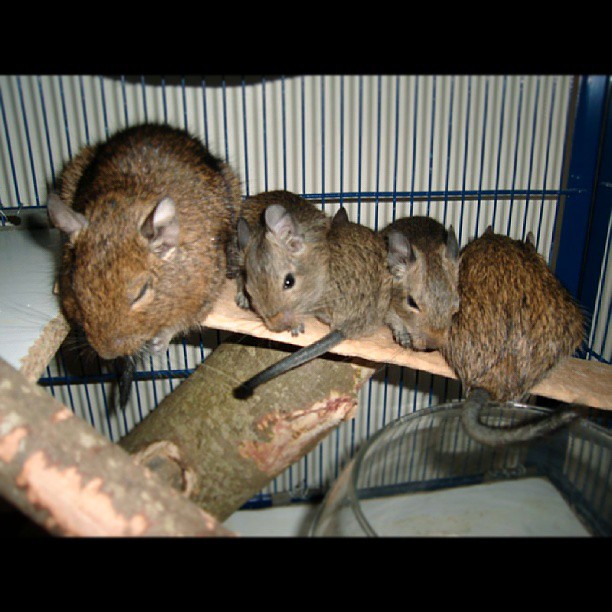This close-up photograph depicts five brown rodents, potentially capybaras or a related species, within a black metal cage featuring blue bars and a white back wall. They are all perched on a slanted wooden board, supported by natural tree branches, some of which show signs of gnawing. The largest rodent, chocolate brown with darker brown stripes and light brown inner ears, is positioned to the left of the image, resting on an angled plank with its eyes closed. Adjacent to it are four smaller rodents, distinguishable by their varied shades of gray and brown. One has its eyes open, suggesting wakefulness amidst its attempt to sleep, while another faces the wall, revealing its black tail. The cage interior includes additional wooden structures, a glass container likely for water, and appears quite compact, facilitating close interaction among the rodents.